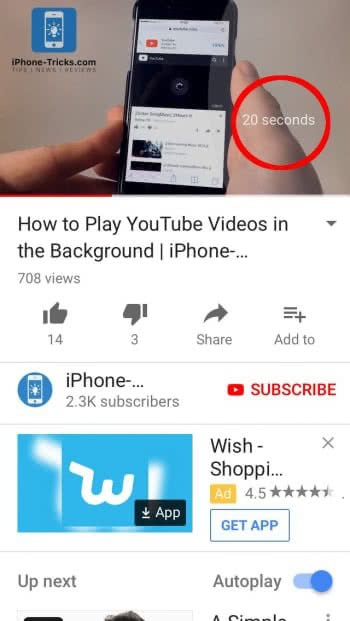A close-up image captures a person holding an iPhone, prominently displaying the screen of the small device. The screen shows a snapshot from iPhonetricks.com, adorned with a distinctive icon—a blue square featuring a white phone and an illuminated light bulb, giving an animated feel. 

In the center of the screen, a red circle with the text "20 seconds" stands out, indicating the duration of a video tutorial. The video title, "How to play YouTube videos in the background on your iPhone," is clearly visible. Below the title, viewer engagement metrics are shown: 708 views, 14 likes, and 3 dislikes. Options to share the video or add it to a list are also present.

Further down, the text iPhone... likely refers to the iPhonetricks channel, which boasts 2,300 subscribers. A prompt to subscribe is visible. Additionally, a blue "W" icon representing the Wish Shopping app with a 4.5-star rating dominates the app section, suggesting users download the app.

In the background, less distinct text hints at upcoming content, indicating this image captures a variety of elements someone might interact with on their iPhone.